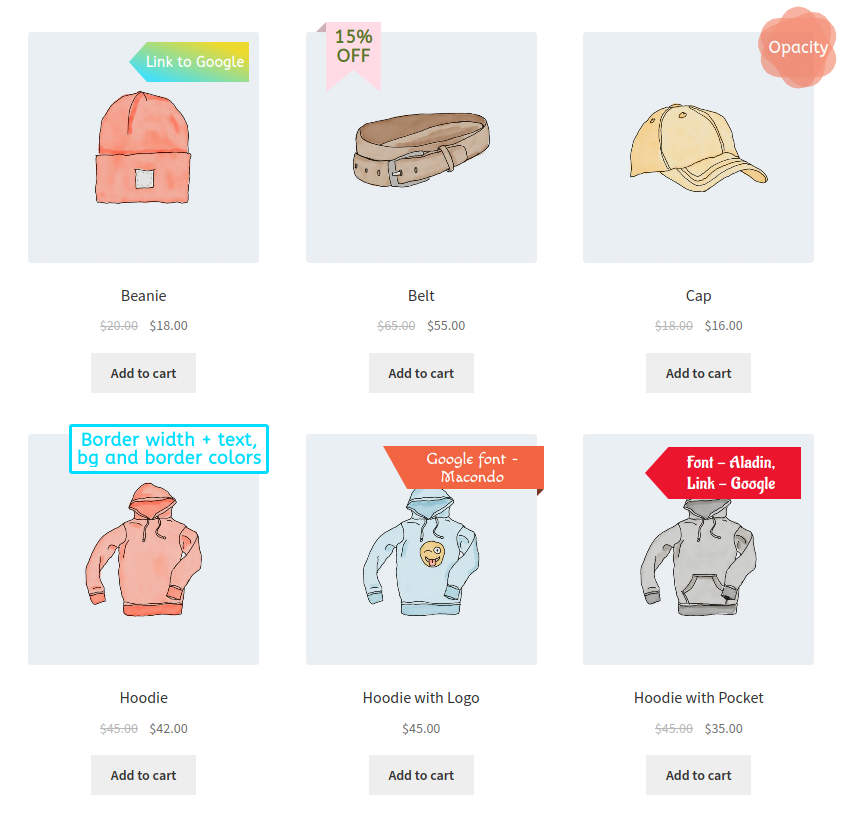The image appears to be a stylized advertisement illustrating various clothing articles, depicted as detailed drawings within six distinct boxes.

1. **Upper Left Box:** This gray box showcases an orange beanie hat featuring a white square at the bottom part. The item's price is $18, and there is an interactive element—an arrow pointing to the left with the text "link to Google." Below the beanie, there is a button labeled "Add to Cart."

2. **Upper Middle Box:** Displayed inside is a belt priced at $55, reduced from its original price of $65. A pink ribbon at the top of the box highlights a 15% discount. There is also a button for adding the belt to the cart.

3. **Upper Right Box:** Featuring a baseball cap in a yellow-brown color, this box is also gray. The text "opacity" is within the box. Like the other boxes, this one includes an "Add to Cart" option.

4. **Lower Left Box:** This box contains an orange sweatshirt, accompanied by detailed text indicating "border width plus text, BG and border colors." This sweatshirt is priced at $42.

5. **Lower Middle Box:** A blue sweatshirt with a smiley face design is placed here. The text "Google font, Macondo" is prominently displayed, and the price for this item is $45.

6. **Lower Right Box:** Not explicitly described, but assumed similar in format to other sections, likely containing another clothing item with descriptive text and an "Add to Cart" option.

Each box not only demonstrates a different type of clothing article but also incorporates graphical texts and interactive elements for online shopping, blending artistic representation with e-commerce functionality.